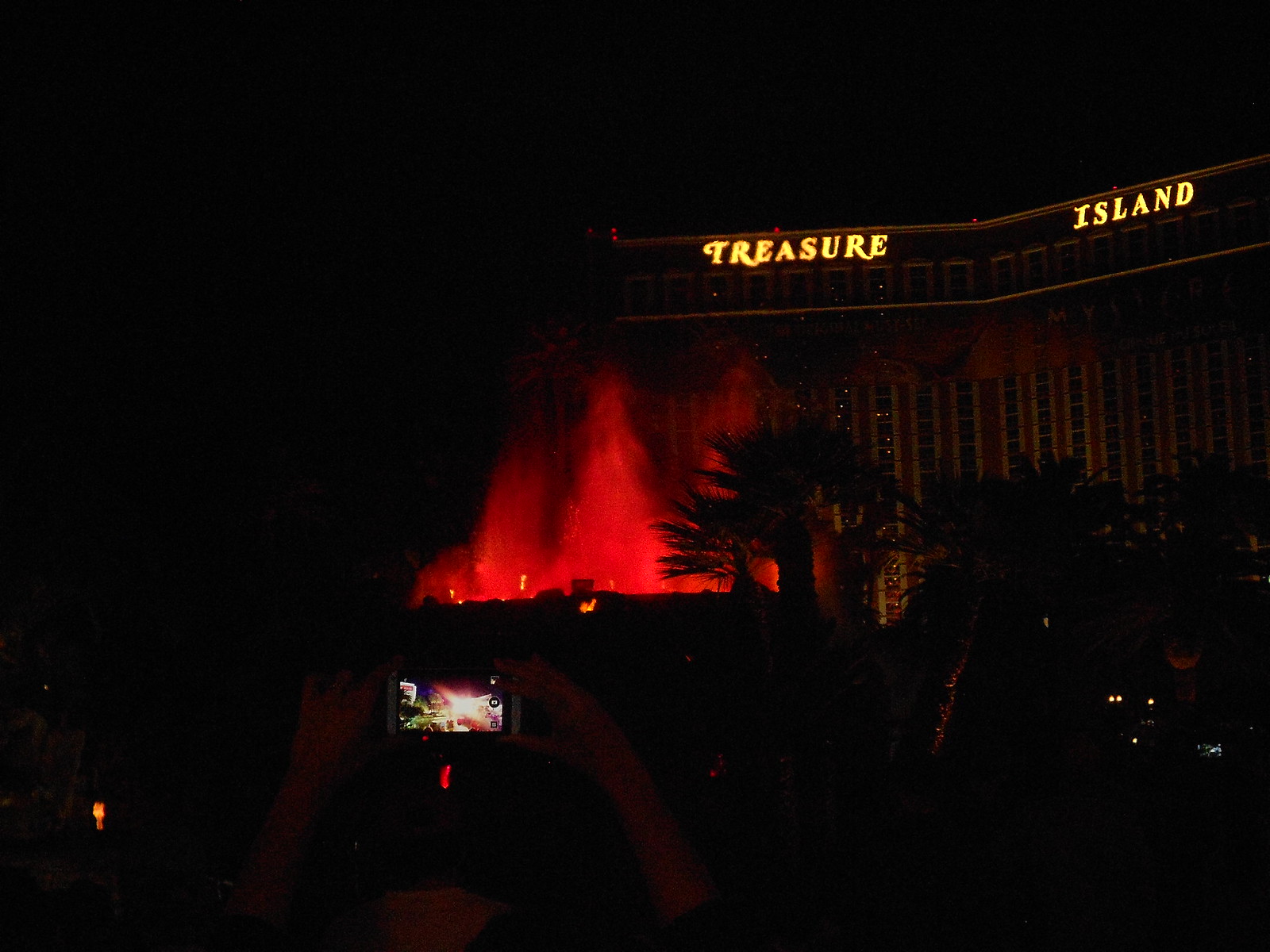This nighttime photograph of Treasure Island captures a vividly lit scene dominated by the neon yellow sign displaying "Treasure Island" atop a tall, multi-story building. The building's unique V-shaped architecture with concave edges is highlighted against the dark night sky, which serves as a stark backdrop. In front of the hotel, a water fountain dramatically sprays water illuminated by red lights, creating an almost fiery effect. Surrounding the fountain are several palm trees, their silhouettes visible against the glow. Additionally, a video camera, its screen illuminated, is positioned near the fountain, apparently recording the captivating display. To the right of the frame, the headlights of various vehicles, including cars and possibly motorcycles, add further intrigue to the scene with one vehicle notably illuminated by a bluish light.